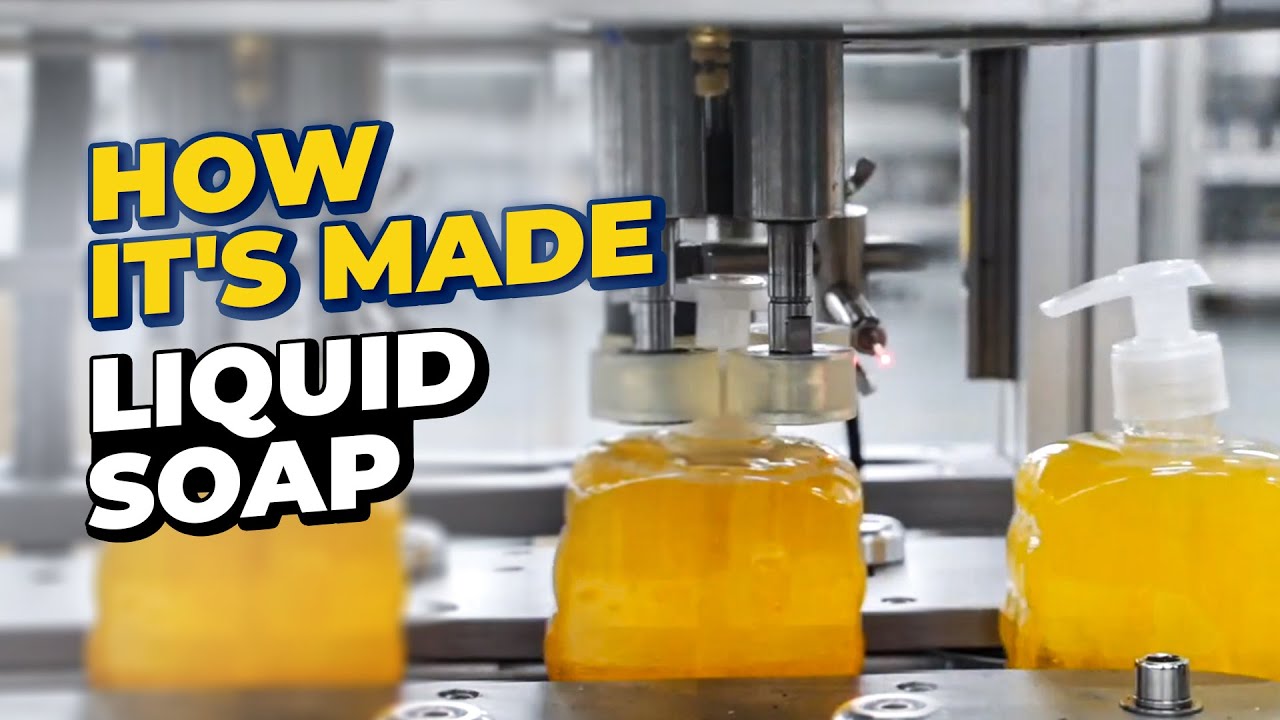This highly detailed photograph captures a pivotal moment in the manufacturing process of liquid soap within a factory setting. Dominating the left side of the horizontally-oriented image is bold, bubble-styled text - "How It's Made" in vibrant yellow with a blue shadow, and beneath it, "Liquid Soap" in white with a black shadow, likely referencing a popular educational show.

Central to the image is a sleek, silver-colored metal machine, integral to the assembly line. Traversing this line are three plastic bottles, each filled with a rich, dark yellow soap reminiscent of marmalade. The bottles are at different stages of cap application: the first bottle on the left remains uncapped, the second bottle in the center is in the process of having its white pump cap applied by a precise metal-automated device, and the third bottle on the right is fully capped.

The capping device is equipped with metal cylinders and rotating white plastic discs at the bottom, meticulously screwing on the caps. This visual encapsulation of the automation process is a testament to the intricate and efficient nature of modern manufacturing.